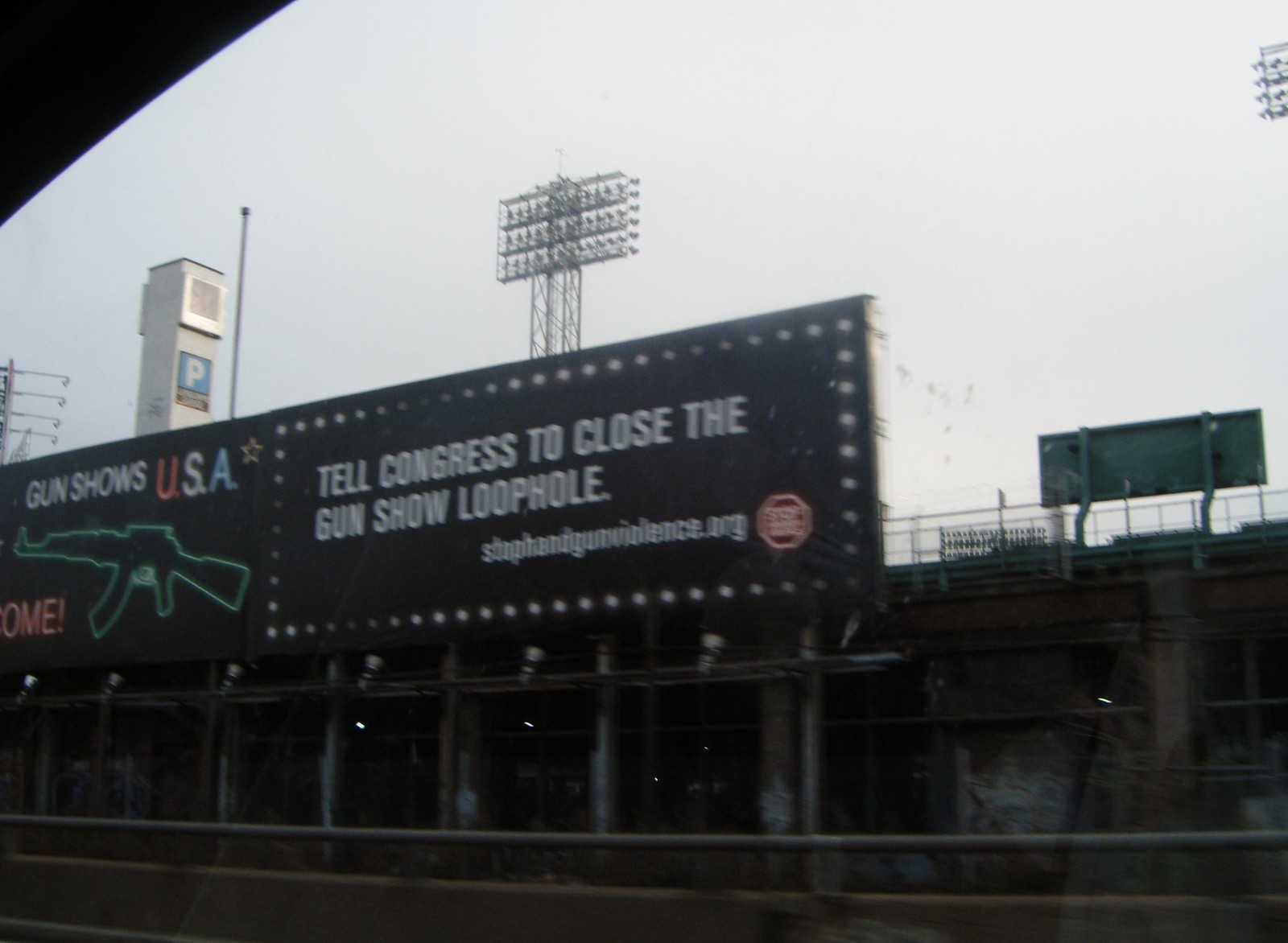A photograph captures a billboard from a moving car, displaying a prominent message outside Fenway Park in Boston, Massachusetts, likely placed there by Senator Ed Markey. The billboard features the text "Gun Shows U.S.A." in red, white, and blue letters, accompanied by a small yellow star in the upper right corner. Below the text is an image of an assault rifle resembling an AK-47. Surrounding some of the text are stars, emphasizing the message: "Tell Congress to close the gun show loophole." At the bottom of the sign, a website is listed: "stopgunviolence.org." Above the billboard, stadium lighting is visible, likely from the ballpark, along with the backs of bleachers and other billboards oriented toward the interior of the park. In the foreground, the car's window is up, slightly reflecting the surroundings, and the picture was taken on an overcast yet pleasant day.